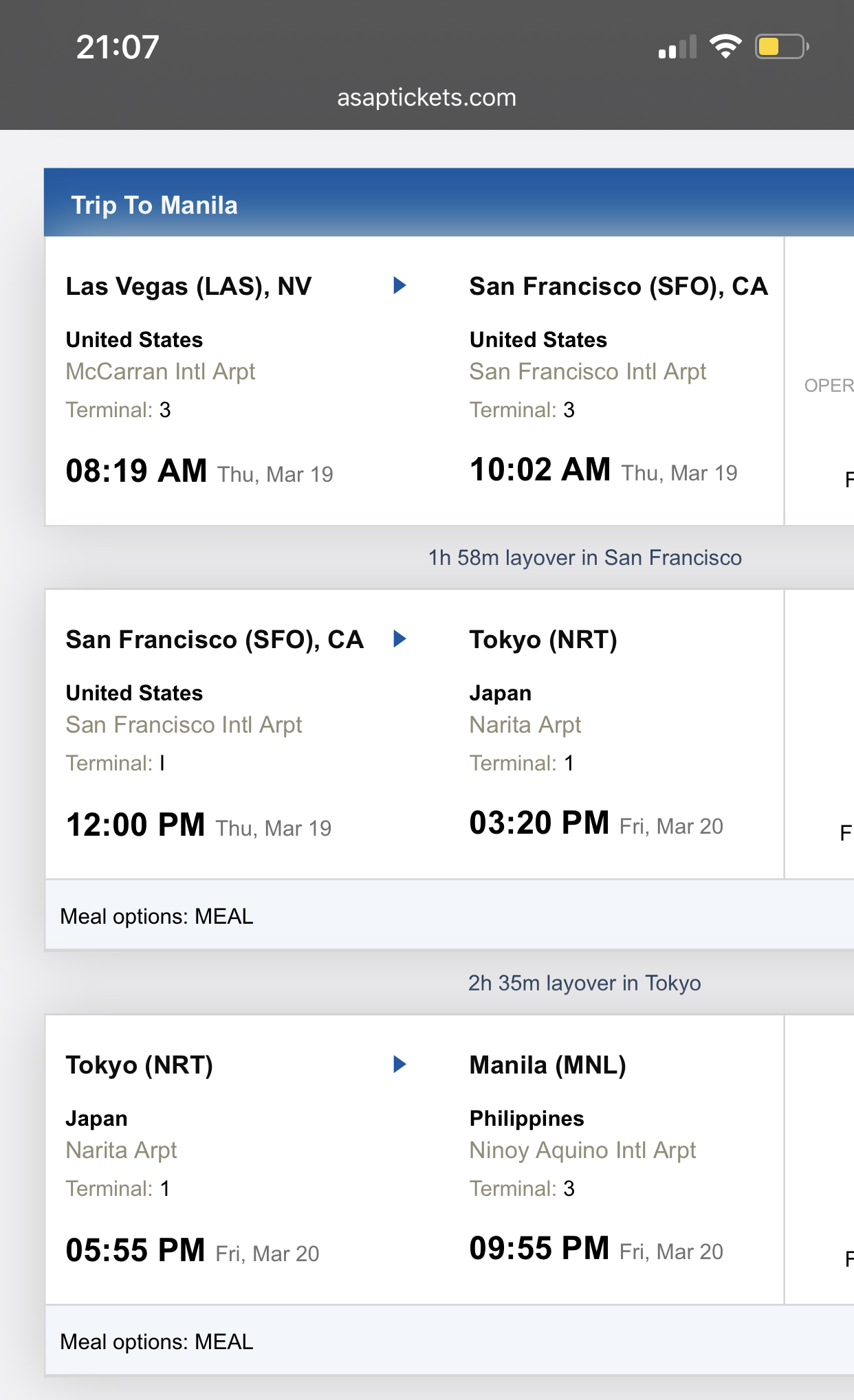The screenshot shows an itinerary from ASAPtickets.com for a trip from Las Vegas, NV to Manila, with several layovers. The top part of the screen displays the current military time as 21:07, along with battery life and Wi-Fi status indicators.

In the middle, there is a prominently displayed box that reads "Tripped in Manila" in white text with a blue border. Below this, an itinerary is laid out in a series of boxed segments:

1. **Las Vegas, NV to San Francisco, USA**
   - **Departure:** McCarran International Terminal 3 at 8:19 PM on Thursday, March 19.
   - **Arrival:** San Francisco at 10:02 PM on the same day.
   - **Layover:** 4 hours and 58 minutes in San Francisco.

2. **San Francisco, USA to Tokyo, Japan**
   - **Departure:** Terminal 1 at 12:00 AM.
   - **Arrival:** 3:20 PM in Tokyo.
   - **Layover:** 2 and a half hours in Tokyo.
   - **Additional Info:** Meal option available.

3. **Tokyo, Japan to Manila, Philippines**
   - **Departure:** Terminal 1 at 5:55 PM.
   - **Arrival:** 9:55 PM in Manila.
   - **Additional Info:** Meal option available.

Each segment box is white with black text, and arrows in blue indicate the direction from one city to the next. Gray boxes underneath each main travel segment show layover information and meal options in light blue text.

On the right side of the screen, there appears to be some cut-off information, potentially showing more details or operator notes for the first trip segment.

Overall, the interface aims to provide clear and structured information about the travel itinerary, with visual aids such as arrows and color-coded details enhancing readability.